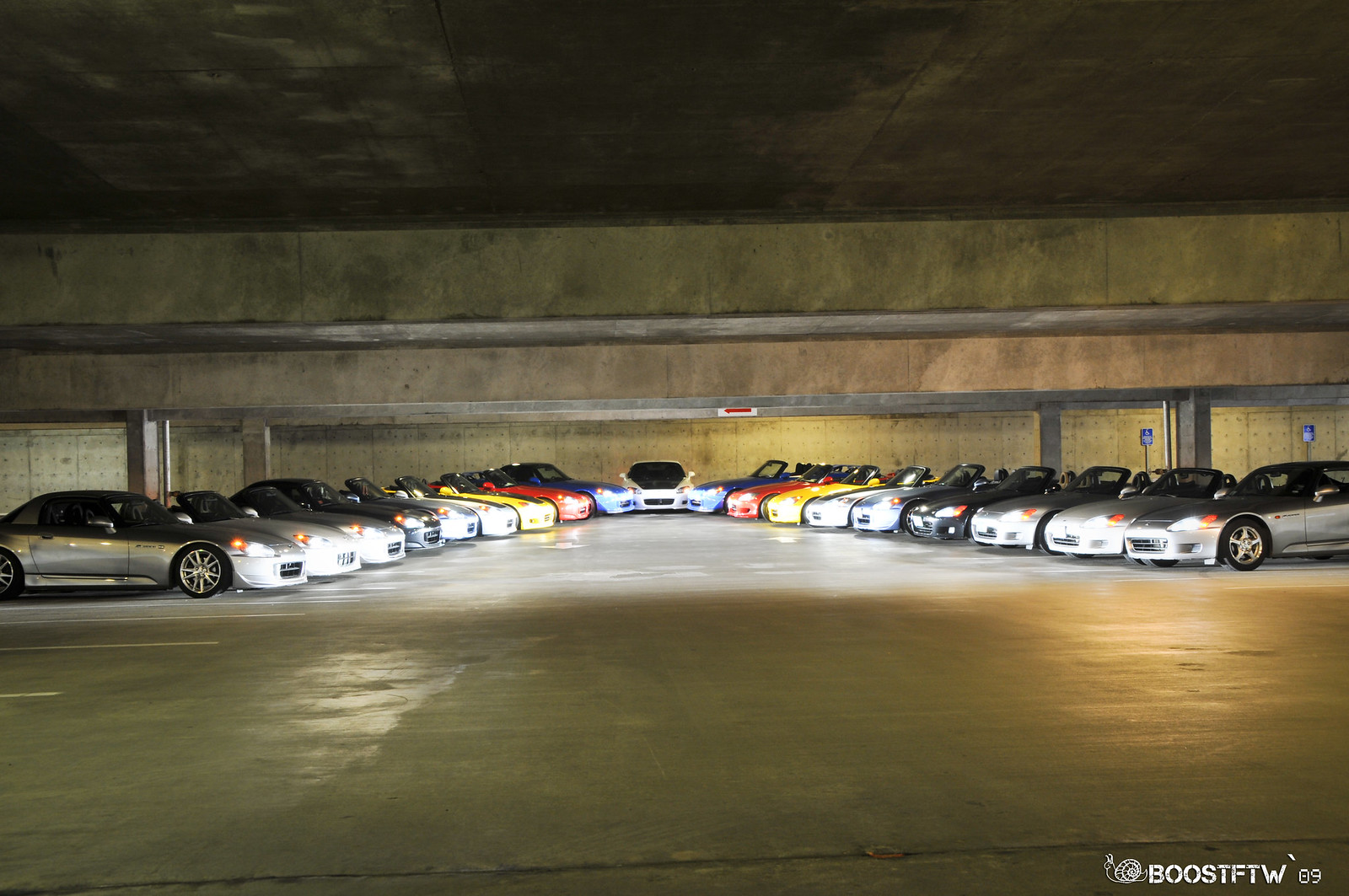In this color photograph, we are inside an underground parking garage that seems to host a car show or meet. The space is dimly lit but is illuminated by the headlights of sporty-looking cars assembled in a precise V-shape formation, with the point of the V furthest from us. The cars, mostly convertibles with many tops down, include a range of colors predominantly featuring silver but also blue, red, yellow, white, and gray. Notably, the car at the center of the V-shape seems to be a Tesla. Handicapped parking signs are visible in the background, and there is a distinctive watermark at the bottom right corner featuring a stylized drawing of a snail next to the text "Boost FTW 09".